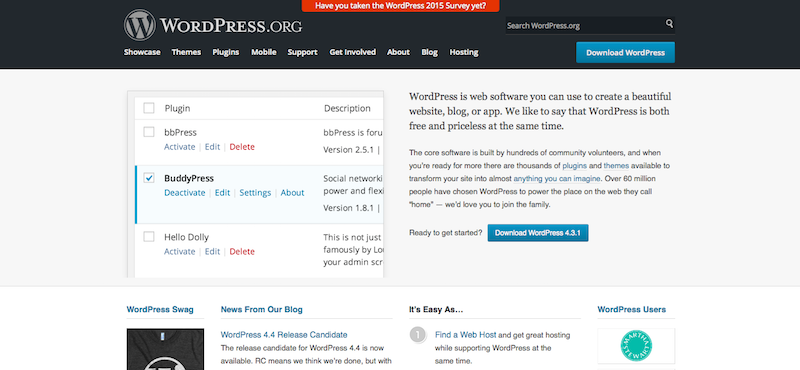The homepage of WordPress.org is designed with a predominantly light gray and white color palette, complemented by a striking black banner at the top. The WordPress logo, featuring a bold "W" encased in a circle with a gray background and black "W," is prominently displayed.

Navigational links within the top banner include "Showcase," "Themes," "Plugins," "Mobile," "Support," "Get Involved," "About," "Blog," and "Hosting." A search bar is conveniently positioned in the top right corner, accompanied by a blue "Download WordPress" button situated just below.

The central section offers a screenshot demonstrative of the software's interface. It describes WordPress as versatile web software ideal for creating various types of websites including blogs and apps. Notably, it emphasizes that while WordPress is free, its value is immeasurable.

Further down, there's an informative segment about plugins, which highlights their role in simplifying the site creation process. Additionally, updates on the platform's latest activities are provided, such as a blog entry about the WordPress 4.4 release candidate.